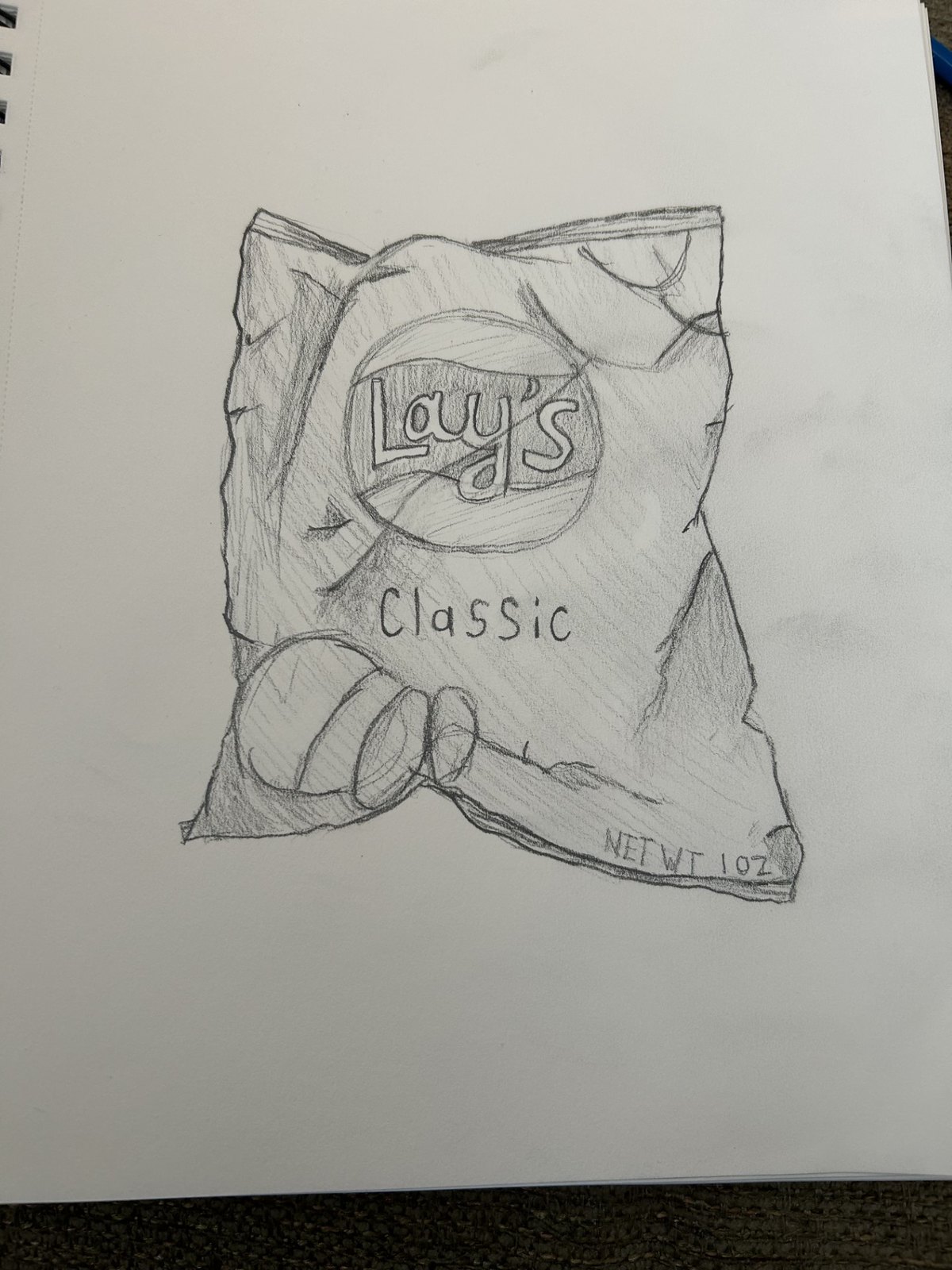This is a detailed photograph of a pencil line drawing depicting a small, crumpled Lays Classic potato chip bag. The black-and-white drawing is done on solid white paper from a spiral notebook, with the characteristic binding spirals visible at the top left corner. The Lays logo, along with the word "Classic," is prominently displayed on the bag, accompanied by an illustration of potato chips. The text "net weight one ounce" is clearly handwritten at the bottom right corner of the bag. The drawing captures the crinkled texture and the sealed top of the bag accurately, with varying intensities of pencil shading giving it depth and dimension. Notably, there is some smearing on the right side, likely from hand contact during the drawing process. The background includes hints of other materials, such as a knitted green surface and a blue element, though the focus remains tight on the hand-drawn chip bag.